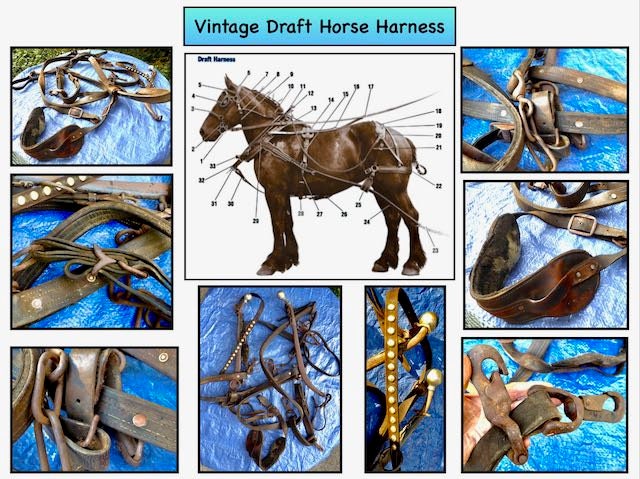The image is a detailed collage showcasing the various components of a vintage draft horse harness. At the center, there is a side profile of a brown draft horse wearing the harness, which is brown leather with some rusted metal components like buckles and attachments. Surrounding the horse are numbers from 1 to 33, arranged clockwise, pointing to different parts of the harness to explain how each part attaches to the horse. Above the horse, the text "Vintage Draft Horse Harness" is prominently displayed in black lettering on a blue gradient background. Around this central image, there are eight close-up photographs of different harness pieces, each placed on a blue tarp, capturing details such as buckles and straps. These smaller images are outlined in black and are set against the same larger white background as the horse diagram, providing a comprehensive view of the harness's structure and components.